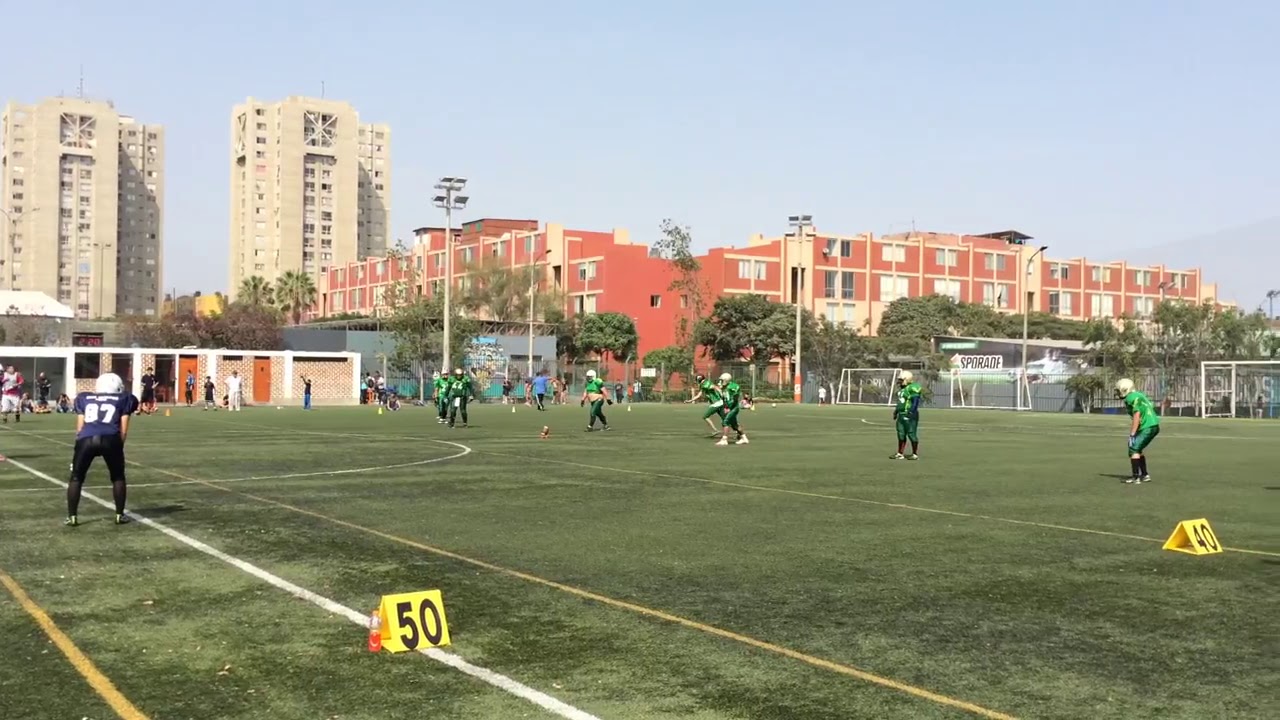This image captures a sunny day at a mixed-use outdoor football field located within a city. The primary focus is on a football practice game with two teams: one team in green jerseys and white helmets, and the other, only partially visible with one player in a purple jersey, black pants, and a white helmet, marked with the number 87. The green team is poised for a kickoff, observable by the placement of the 50 and 40-yard yellow markers on the field. In the background, there are various structures, including a prominent light burnt red brick apartment building with numerous windows, and two high-rise gray towers with a plain cement color, also covered in windows. The sky is clear and blue, indicating pleasant weather, while the field itself is marked for both football and soccer, evident from the three soccer goals positioned at the far right end. Sparse players and a coach are seen on the sidelines, adding to the dynamic yet practiced atmosphere of the scene.